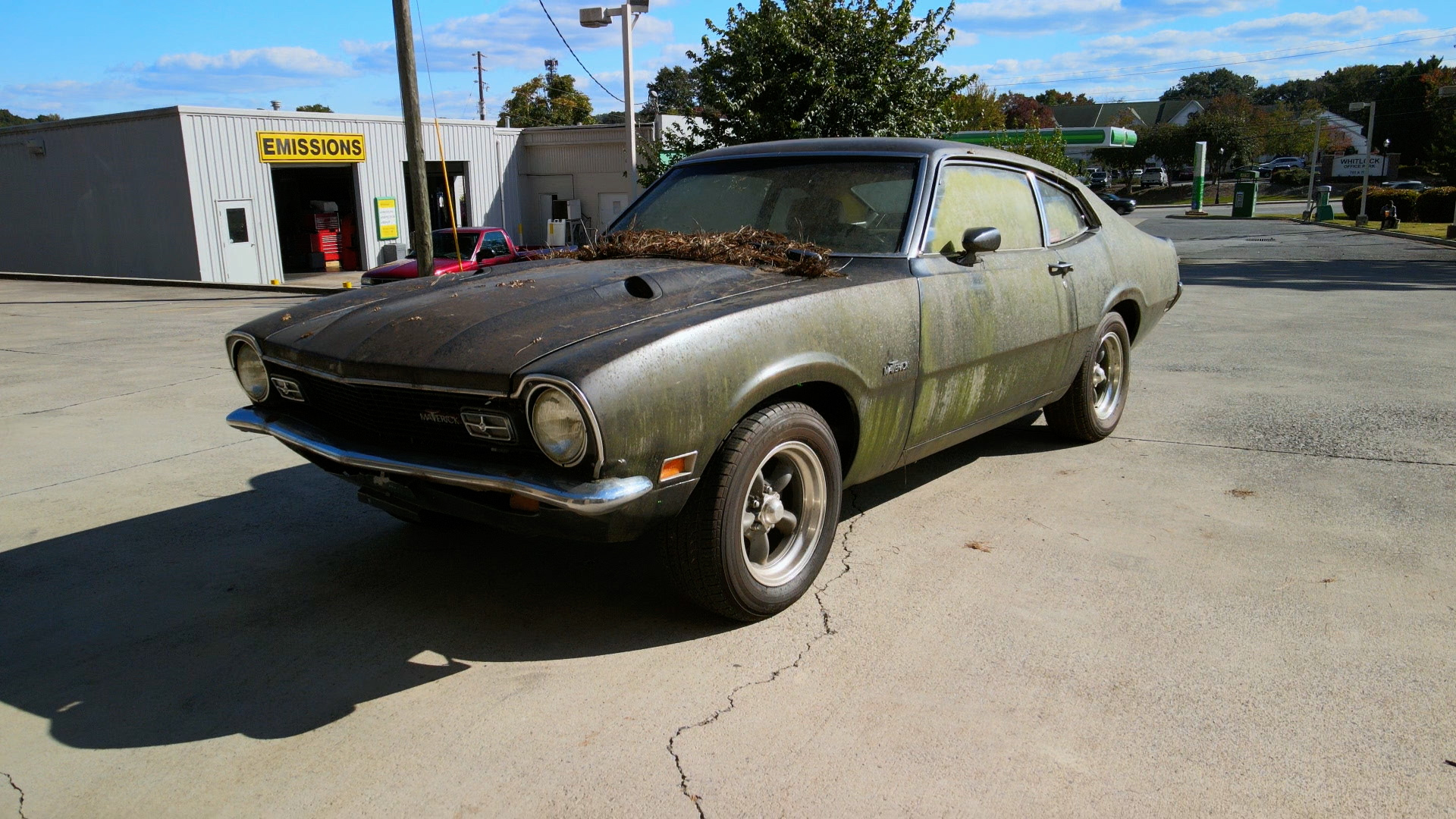In the outdoor image, an old, rusted car with weathered green paint sits stationary on a cracked concrete surface. The car appears neglected, adorned with a layer of dead leaves on its roof and moss overgrown on the dirty windows, indicating it hasn't been moved in a long time. The vehicle, which has black tires and silver wheels, shows significant signs of age and disuse. To the left, a building with a golden sign reading "ADMISSIONS" in black, capital letters stands prominently. Adjacent to this is a flat-roofed garage with a door labeled "EMISSIONS." A nearby horse trailer and green rooftop—reminiscent of those typically found on BP gas stations—add to the background details, alongside light poles, green trees, and bushes under a colorful sky streaked with blue, purple, pink, white, and gray clouds.